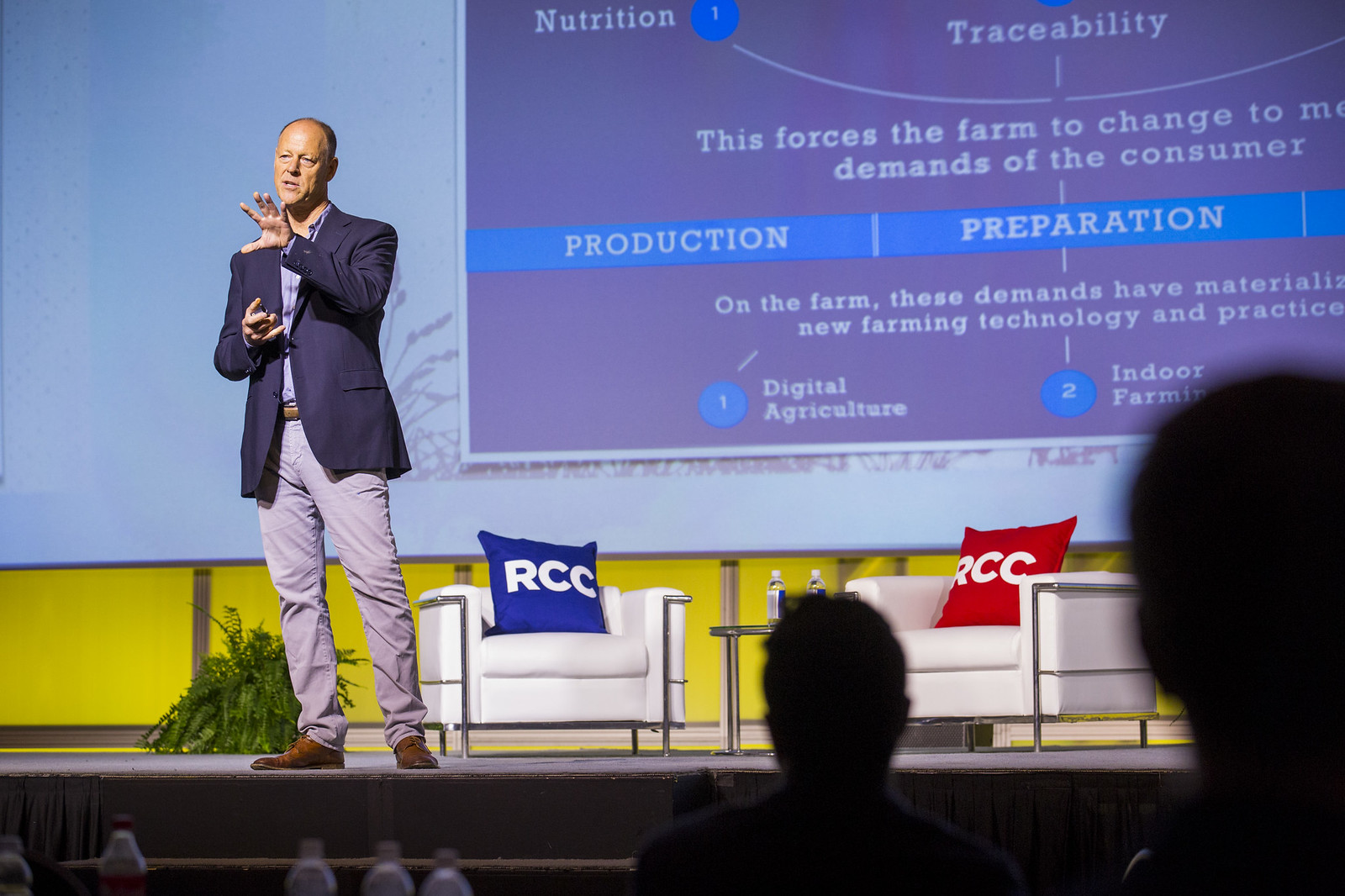A balding, white man stands confidently on a stage in a large indoor venue, addressing an attentive audience. Dressed in a dark blue blazer, light blue button-up shirt, beige khakis, and brown shoes, he gestures animatedly with his left hand extended and fingers spread, while his right hand rests near his waistline. 

In the foreground, the silhouettes of audience members' heads are visible, emphasizing the engaged crowd listening to him speak. Bottles of water or other drinks are placed in front of the stage, presumably for the attendees. 

Behind the speaker, there are two white chairs, each adorned with a square pillow bearing the white capital letters "RCC"—one pillow is blue, and the other is red. A coffee table between the chairs holds two bottles of water. 

A large projector screen dominates the background, displaying a presentation slide with text focused on nutrition, traceability, and the evolving demands in farming technology. The slide reads: "This forces the farm to change to..." and continues with keywords and phrases like "digital agriculture," "indoor farming," "production," "preparation," and "on the farm these demands have materialized," indicating a discussion on new farming practices and technology.

The scene is reminiscent of notable public speakers like Steve Jobs, capturing a moment of dynamic engagement and informative discussion.